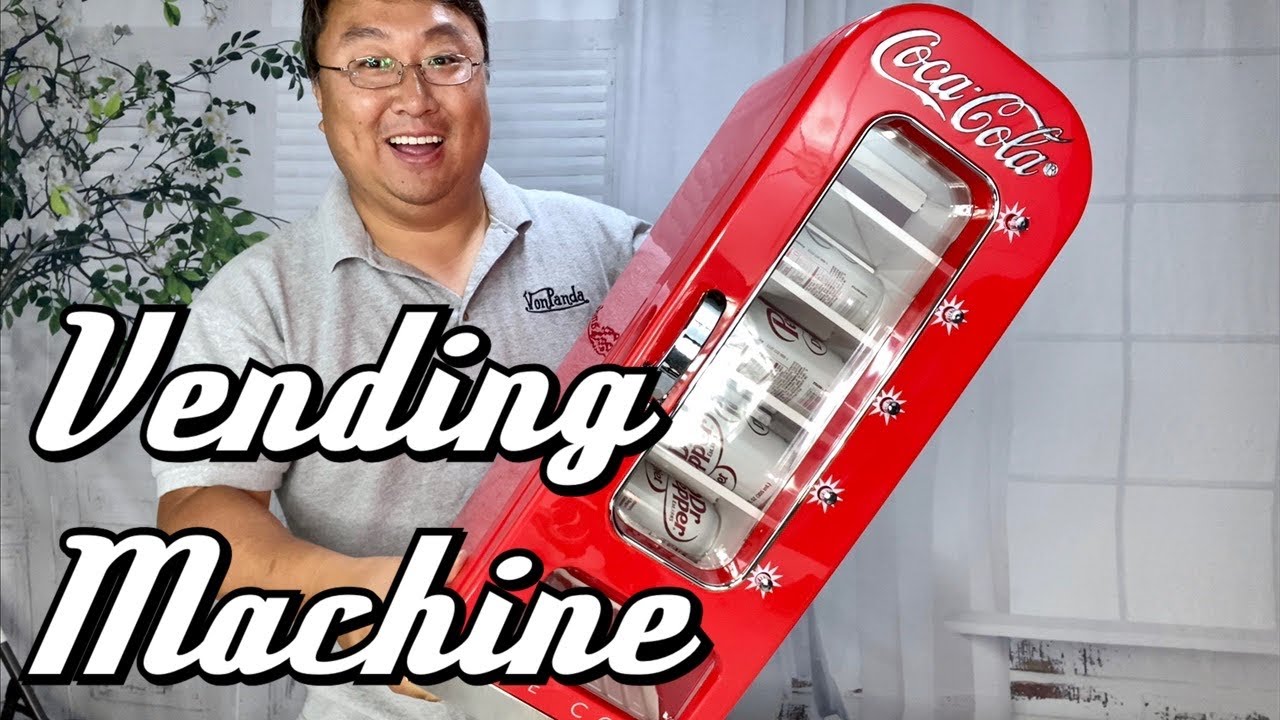In this detailed image, an Asian man with round glasses and a wide-open smile, showcasing his happiness, is captured from the waist up. He is dressed in a light gray polo t-shirt and holding a retro-designed Coca-Cola mini fridge. This vibrant, metallic-red fridge proudly displays the Coca-Cola logo at the top in bold, silver letters. The fridge features a glass door with a small silver handle, revealing a stash of Dr. Pepper cans inside. The background consists of a white wall with a window adorned by white blinds, and to the man's left stands a tall, lush green plant. On the left side of the image, in large white font with black shadows, the words "Vending Machine" prominently appear, adding to the nostalgic feel of the scene.